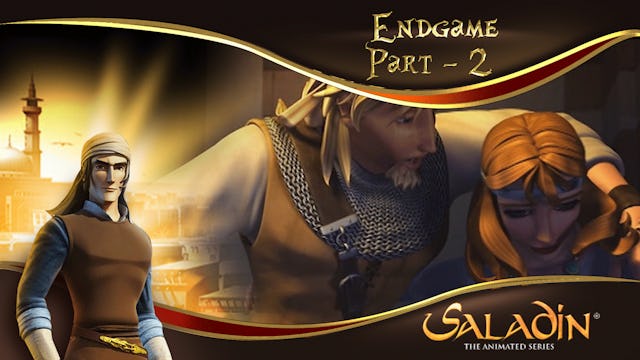This detailed image is likely a snapshot or an advertisement for a video game, labeled "Endgame Part 2" in stylized, old-time-looking gold font at the top. The backdrop features a dark brown and black background, with swirling designs marking the title and the bottom text. The bottom text reads "Solid Den" in gold letters with "The Animated Series" underneath in small, white, all-capitalized letters.

Depicted on the right side of the image is a blonde-haired, light-skinned man wearing chainmail around his neck, a brown leather strap across his chest, and a tan vest over a cream-colored shirt. He has a blonde goatee and shoulder-length hair. The man is consoling a light-skinned woman with shoulder-length red hair that hangs down and includes bangs. She appears to be looking downward.

On the left side of the image, another man stands alone in the foreground. He is light-skinned, wearing a cream-colored turban that hangs down his back, a brown vest or robe, and a blue shirt with the sleeves rolled up. He also has a brown belt with gold embossments and a sword sheath at his hip.

The background of the image reveals a city with a sunset glow and a prominent tower rising above the buildings, all objects aligned at right angles, adding a structured aesthetic.